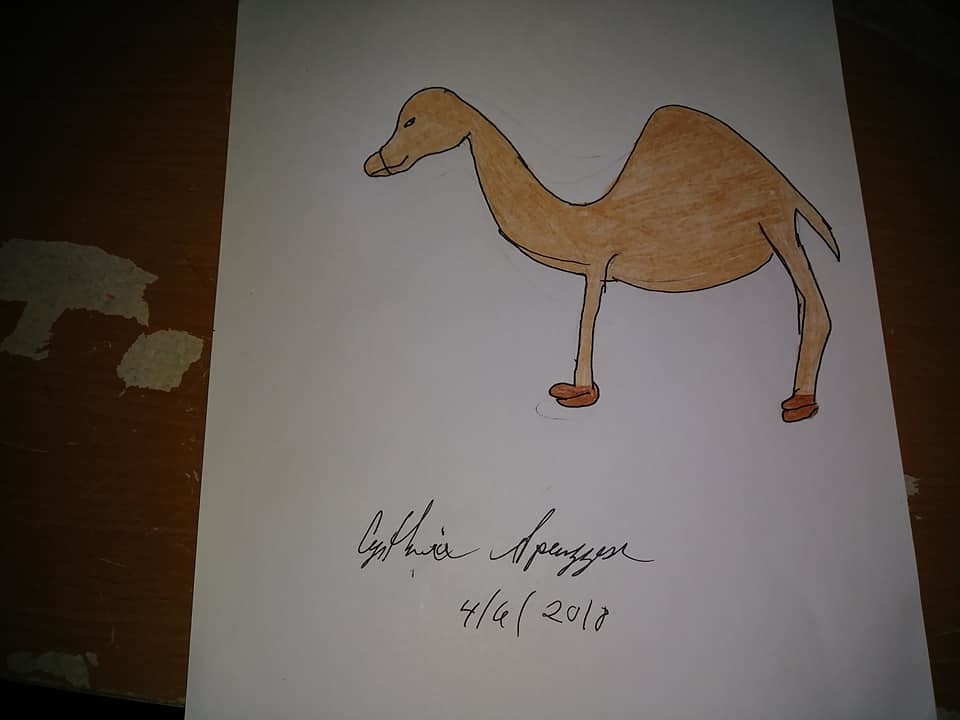In this slightly dim, low-light photograph, a hand-drawn image on a piece of standard white printer paper takes center stage. The drawing depicts a rather whimsical brown camel, situated atop a brown table that shows signs of wear, with noticeable white, bald patches on the left-middle side of the frame. These patches suggest the table has sustained some paint loss over time.

The camel, although endearing, is quite crudely rendered with several anatomical quirks. Its neck is oddly elongated, bearing a striking resemblance to a boa constrictor rather than a camel's usual stout structure. From the elongated neck upwards, the camel sports a jovial smile and an eye that appears to be plotting. The face includes a suggestive line through the muzzle area.

The camel's body is light tan, with a prominent single hump on its back. It has two visible legs, one foreleg and one hind leg, each ending in a brown, two-toed hoof. The body extends back to a very short, stubby tail, and a part of another leg with a similarly rendered two-toed foot is visible along the stomach and neck area.

In the bottom right corner of the drawing, a signature reads "Cynthia Appazin" in cursive, alongside the date 4-6-2018, marking the creator and the date of completion of this charmingly imperfect sketch.